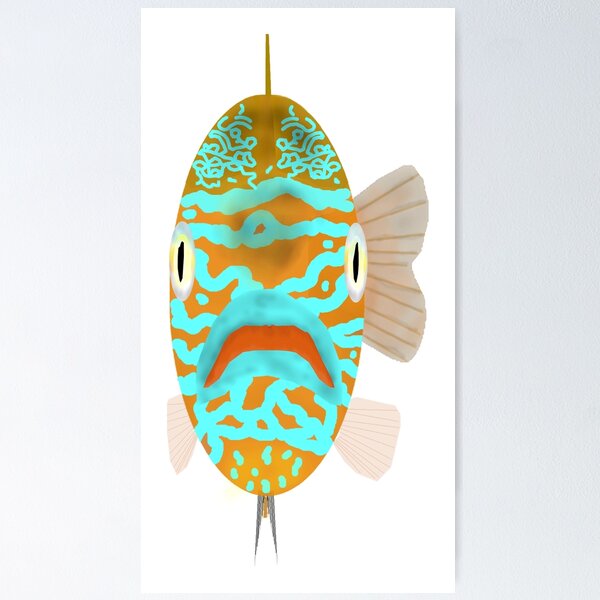A front-facing drawing of a multicolored fish is centered on a white canvas against a gray background. The fish's body is a large, elongated oval, primarily in a yellowish-brown or yellowish-orange hue. Distinct blue or teal squiggly stripes and spots pattern the body, creating a vivid contrast. The fish has prominent eyes on either side of its head, which are white with light yellow accents. The mouth is a bright aqua color. Its tail fin, resembling a heart shape, is white with brown stripes and extends to the right. Additionally, two small fins on the bottom left and right share the same white and brown-striped pattern, while gray fins appear on the lower part of the body. A single large fin protrudes from the top of its head. The artistic representation suggests the fish is slightly dried out, emphasizing its textured appearance.